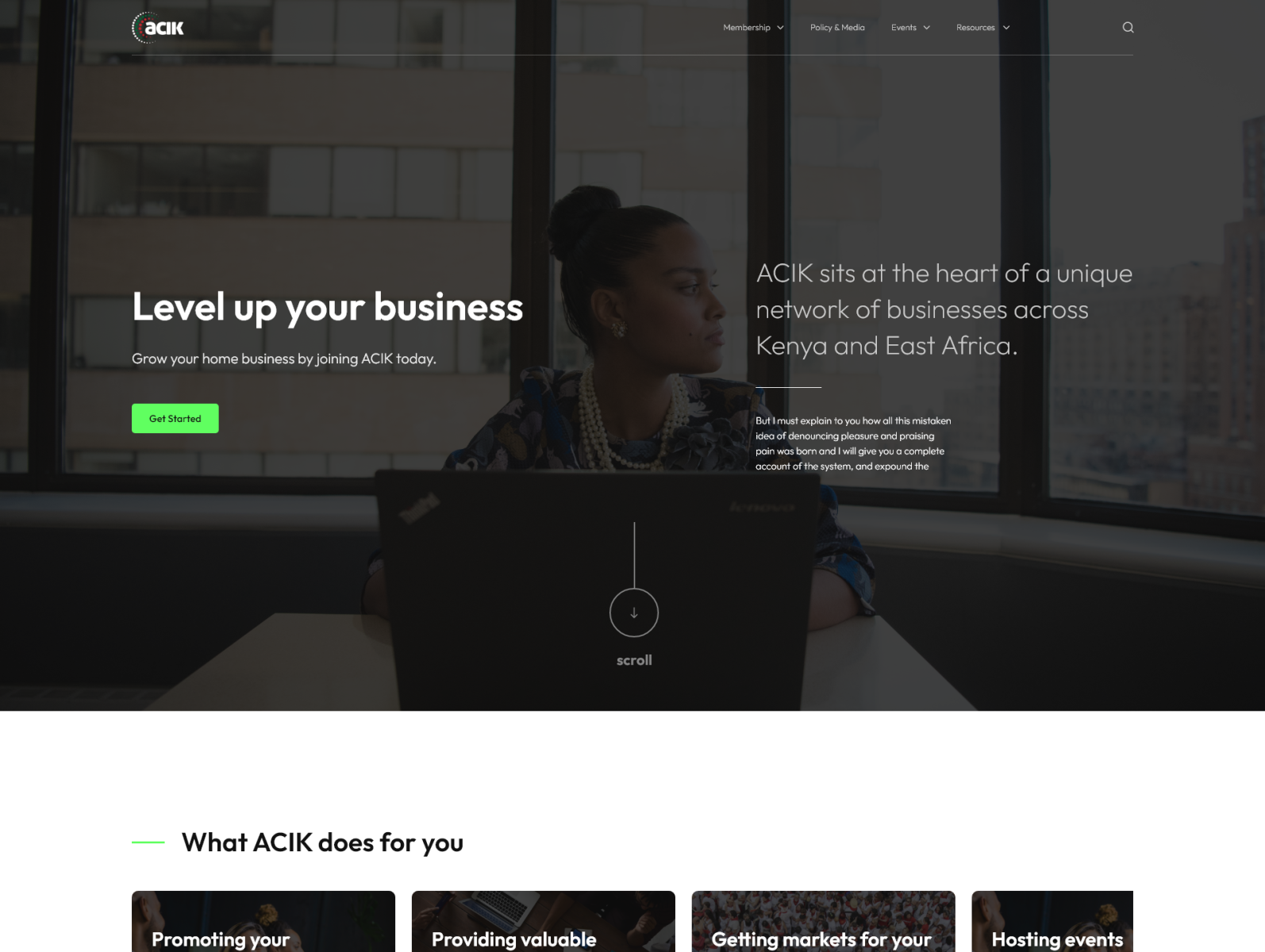The image prominently covers most of the page and features a serene yet dynamic scene set against a grayed-out, transparent background. At the center of the composition sits an African woman with her rich, black hair styled in a bun, gazing contemplatively off to the side. She is adorned in elegant white pearl necklaces and wears a vibrant, intricately-patterned shirt in blue and orange hues traditional to African attire. The backdrop showcases a modern office environment with large square and rectangular windows that provide a glimpse of an urban cityscape filled with office buildings.

In the upper left corner, bold white letters spell out "ACIK" next to a semi-circle logo in red, white, and blue, underlined by a faint white line. The upper right corner displays various menu options, but they are too small to decipher clearly, although a magnifying glass icon suggests a search function.

Central to the picture, on the left, large white letters announce, "Level up your business," followed by the slogan, "Grow your home business by joining ACIK today." Directly below this message, a bright green box with black text invites viewers to "Get Started."

To the right of the woman, another text block reads, "ACIK sits at the heart of a unique network of businesses across Kenya and East Africa." Below this is a paragraph of text in white, but it is too fine to read. A thin white line extends over the laptop in front of the woman, ending at a white circle with an arrow pointing downwards, accompanied by the word "Scroll" in white.

Further down, a subtle blue line runs across the image, where black letters to the right state, "What ACIK does for you." Under this line are four images partially cut off, each with a caption in white letters. From left to right, they read: "Promoting your," "Providing valuable," "Getting markets for your," and "Hosting event." However, the truncation of both pictures and text makes it difficult to discern the full context of these images.